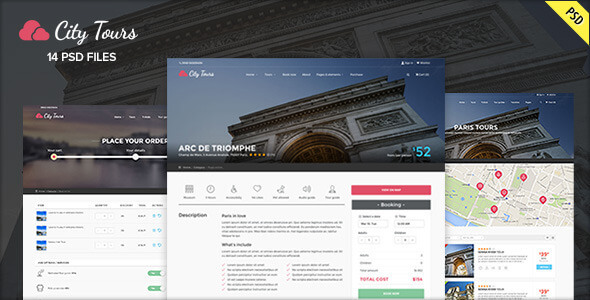This image is a visually striking advertisement for a company called City Tours. It appears to be a screenshot, given its long rectangular shape resembling the dimensions of a desktop monitor. Dominating the upper left-hand corner of the image is an illustration of two small clouds, tinged with a pinkish-red hue. Adjacent to these clouds, the company name "City Tours" is elegantly displayed in white cursive text. Directly beneath the logo, the text "14 PSD files" is prominently featured, indicating the inclusion of 14 Photoshop files.

The background layer of the image showcases a semi-distorted, darkened, and obscured representation of grand architecture, possibly reminiscent of structures found in Rome or France. The architectural elements are captured from an upward angle, giving an impression of stone buildings, though specific details are deliberately blurred to keep the focus on the main content.

Overlaying this backdrop are three distinct images, likely screenshots highlighting various programs or services offered in the City Tour package. These overlaid images serve to provide a glimpse into the diverse experiences or itineraries available through the company's offerings. The overall composition blends aesthetically rendered graphical elements with informative content, designed to entice potential customers to explore City Tours.